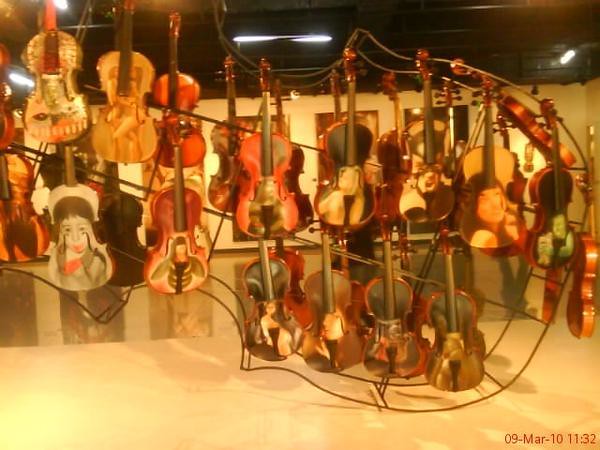The image depicts a striking art installation featuring over 20 violins suspended from a large, wireframe sculpture shaped like a violin. The sculpture leans towards the top left of the frame, creating a dynamic visual composition. Each violin showcases unique designs, including artistic depictions of people and animals, adding an eclectic and intriguing element to the display. The backdrop includes a partially visible wall adorned with paintings and a platform beneath the sculpture. The scene is illuminated by white lights set against a black ceiling, providing a contrasting backdrop to the colorful violins. A timestamp reading "09 Mar 10 11:32" is visible in maroon text at the bottom right of the image.